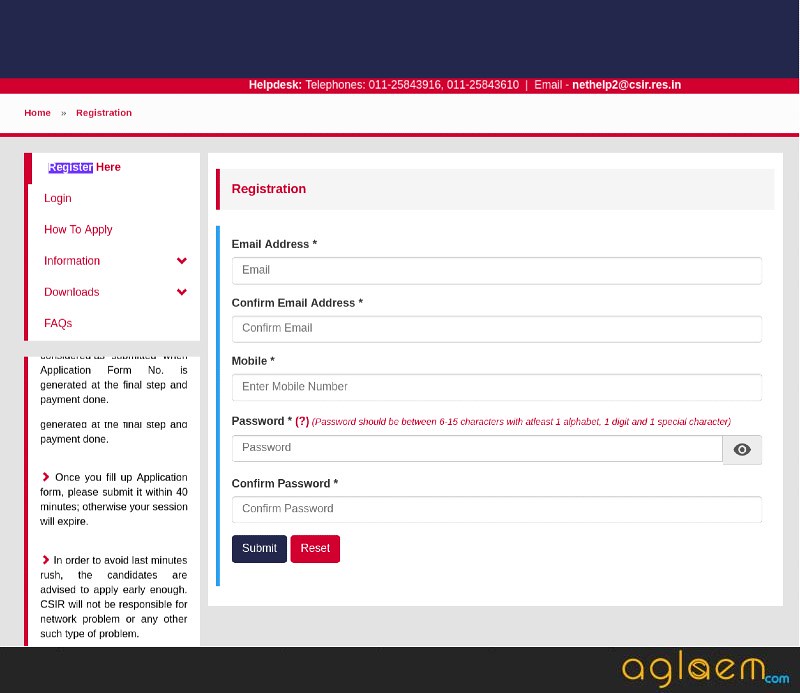Screenshot of a User Registration Page

The image showcases a user registration page with a structured layout and distinct color scheme. At the top, there is a dark blue horizontal bar, followed by a thin red bar beneath it, which prominently displays "Help Desk Telephones" along with a contact number and email address, all in white text. Below this section, on the left side in a white area, are two red links labeled "Home" and "Registration." Another thin red bar divides this area from the main content below.

The main section of the page has a grey background and includes two main components: a sidebar on the left and a registration form on the right. The sidebar features a vertical list of buttons for different actions and information: "Register Here," "Log In," "How to Apply," "Information," "Downloads," and "FAQs." Notably, the "Information" and "Downloads" buttons are drop-down menus.

The registration form on the right is topped with a grey bar that has the word "Registration" in red text. The form itself is white and contains fields for "Email Address," "Confirmed Email Address," "Mobile," "Password," and "Confirmed Password," each marked with an asterisk to indicate required information. At the bottom of the form are two buttons: one blue "Submit" button and one red "Reset" button.